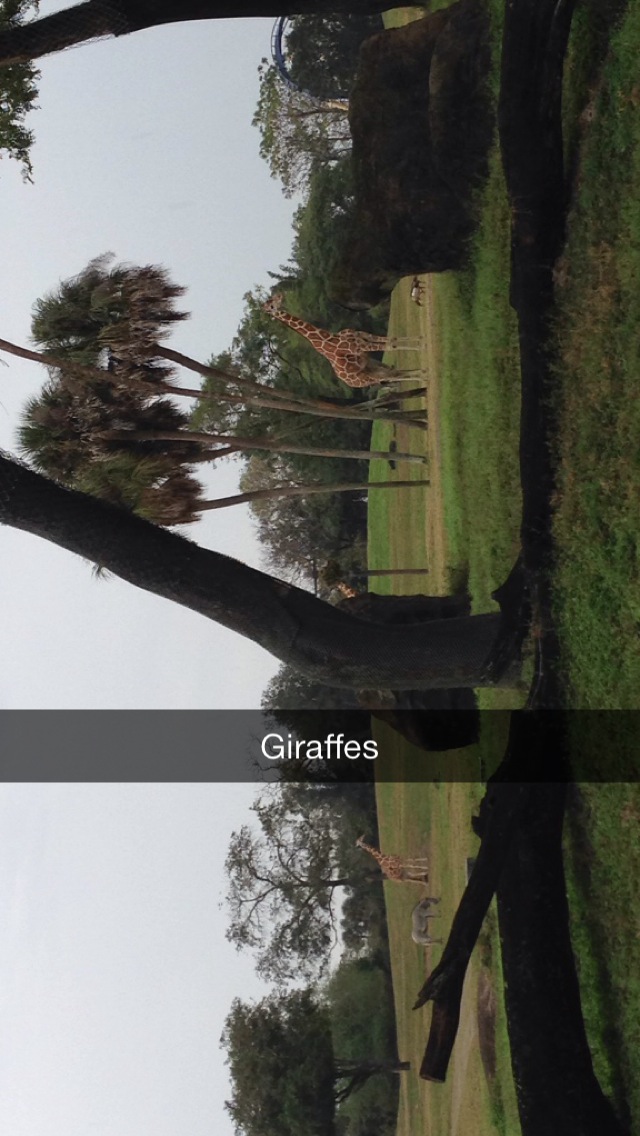This horizontally-oriented rectangular photograph is displayed sideways, requiring viewers to turn their heads to the left to properly view it. The scene seems to be set in a sanctuary, wildlife park, or zoo rather than the wild, featuring two giraffes. In the foreground, a taller giraffe donning an orange coat with dark orange-brown spots stands beneath a trio of palm trees, against what appears to be a well-manicured, grassy area that resembles a golf course. A smaller, baby giraffe is positioned to the left of the taller one, accompanied by a small, unidentified gray animal, possibly a goat. The background includes sparse trees and some scattered foliage, with a light blue sky overhead that is somewhat overcast. A translucent black banner with white text spelling "giraffes" stretches across the middle of the photo, suggesting it might be from Snapchat.